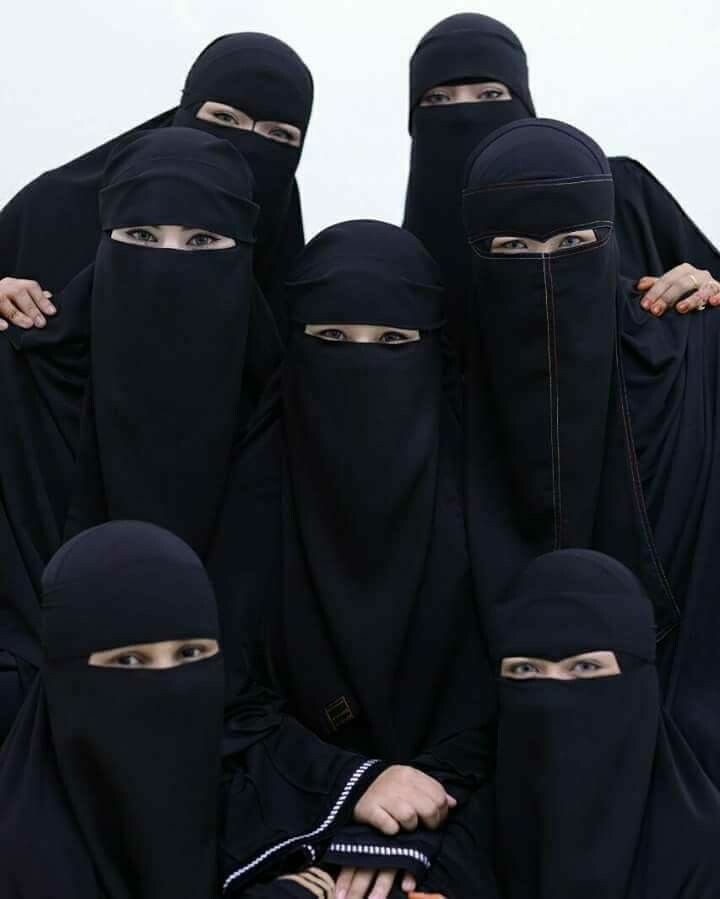This is a color photograph of seven women wearing black burqas, each with only a small slit revealing their eyes. The women are posed in three tiers: two women at the front whose visibility is limited to their heads, three women slightly above them with one centrally positioned, and two women forming the topmost row. A hand is placed on the shoulder of each woman, while the woman at the center of the middle row has her hands folded over each other, showcasing some light-colored embroidery on her sleeves. The background is a very light sky blue, suggesting an outdoor setting. The burqas, which have hood-like coverings connected to the rest of the garment, also feature some instances of top stitching or embroidery. One woman’s hand is particularly noted for its visibility.